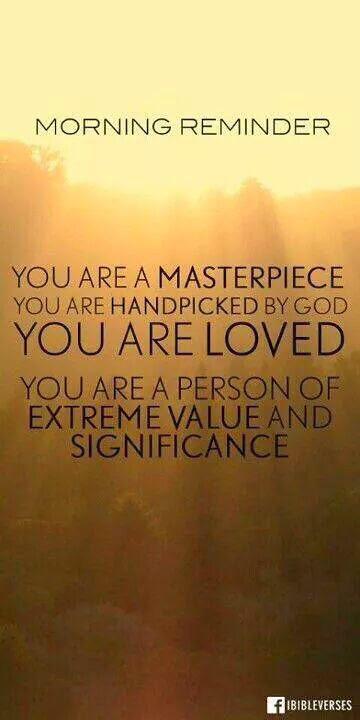The image resembles a book cover or a digital screen, bearing a motivational message. At the top, "Morning Reminder" is prominently displayed in large, blue, all-capital letters against a sunlit, blush-colored sky that transitions into an aerial view of a forest with indistinct, blurry trees. Below, the following text appears in varying sizes and styles in blue all-capitals: 

- "You are a masterpiece" (with "masterpiece" in bold)
- "You are handpicked by God" (potentially with "God" in a different color)
- "You are loved" (in large letters)
- "You are a person of extreme value" (with "extreme value and significance" in bold)

At the bottom right corner, there's a small "F" Facebook icon followed by "Bible verses." The background features a color gradient from light beige, glowing with a sunlit effect, fading into darker shades of chestnut brown, creating a warm, serene atmosphere suited for a social media post.